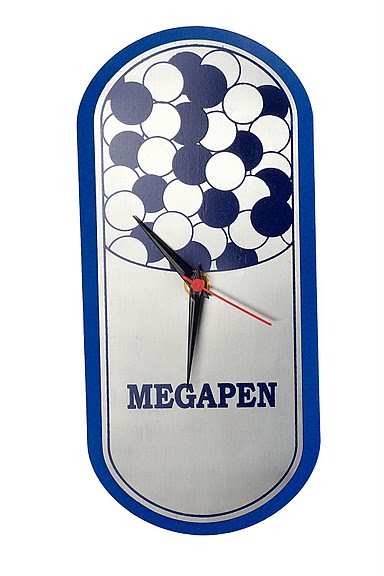The image showcases a clock designed in the shape of a pill, promoting the Megapen product, a medicine for bacterial infections. Predominantly white with a navy blue or electric blue border, the clock features an oval, pill-like design. Inside, it displays a mix of white and navy blue circles, suggesting medication capsules. The clock hands are black, with a red second hand adding a striking contrast. Centered on the lower part of the pill shape, the name "Megapen" is displayed prominently in capital letters in navy blue. The clock's time reads approximately 10:32, and the bottom part has a subtle silver appearance, enhancing the overall design.